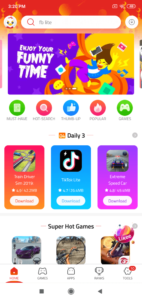This screenshot from a cell phone depicts a rather chaotic and blurry interface, making much of the text difficult to decipher. At the top, there's a red banner showcasing a city skyline with several crescent moons interspersed. Beside the search bar, an avatar resembling an anthropomorphized chicken is visible, though the text within the search bar itself is illegible.

Beneath the banner, a vibrant purple and yellow illustration catches the eye, depicting a person seemingly falling from the sky. The character wears a broad smile and flashes a peace sign with their left hand while clutching a cell phone in their right hand. To the left of the image, text reads, "Enjoy your funny time."

Below this illustration, there are several interactive icons: a green icon with a white piece of paper labeled "must have," a red circle with a white magnifying glass labeled "hot search," a blue circle with a white thumbs-up labeled "thumbs up," and a red circle with a white flame labeled "popular." Additionally, a green icon featuring a white video game controller reads "games."

Further down, under the heading "daily three," three smaller icons are visible. The one on the left is too blurry to identify. The middle icon represents TikTok, and the right icon seems to depict a driving game. Unfortunately, the text beneath these icons is too obscure to read.

At the bottom of the screenshot, a section titled "super hot games" is partially visible, though the detailed contents remain unclear. The overall impression is of a busy, colorful interface filled with various entertainment options and search functionalities.